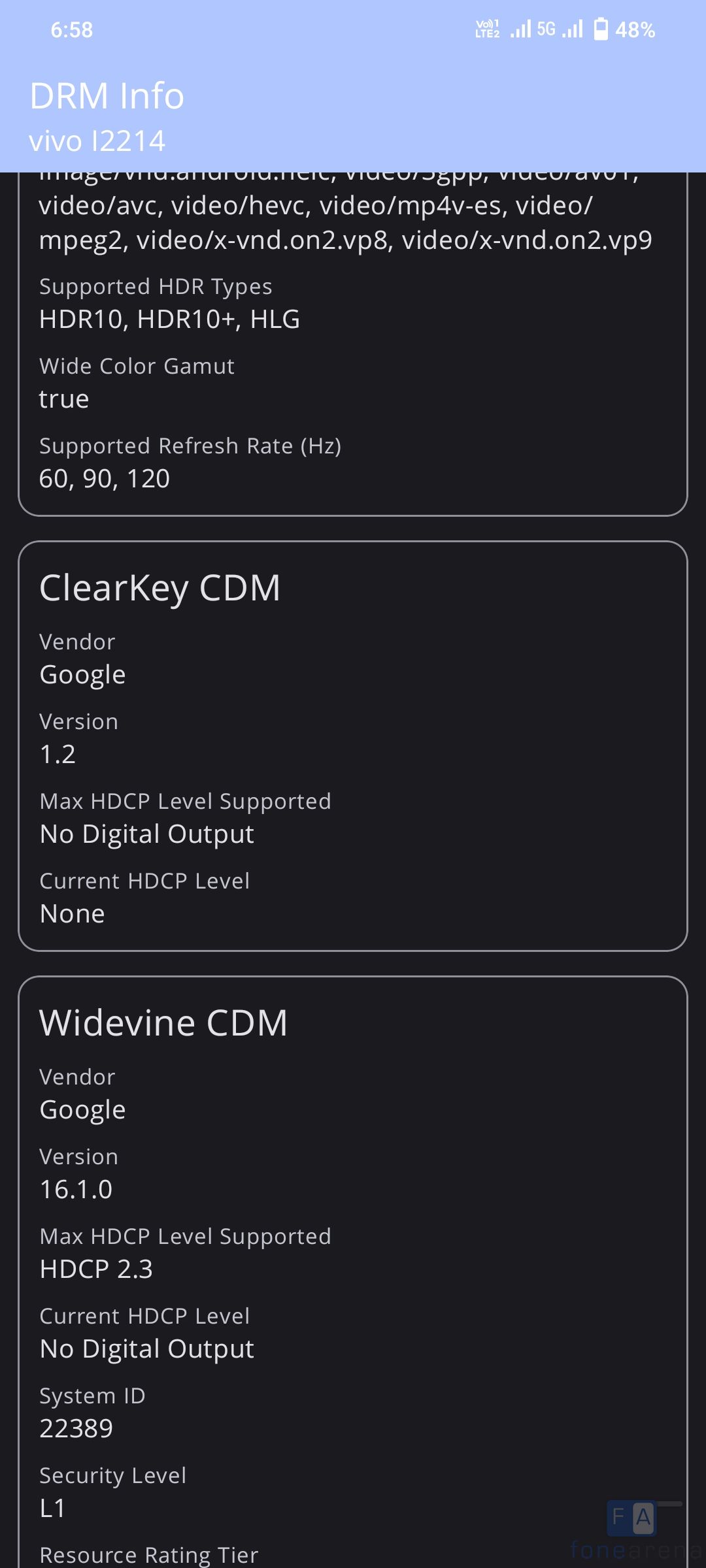At the very top of the image, there's a light blue rectangle displaying the time as 6:58. On the right side of this rectangle, the battery icon indicates a 48% charge, and a "5G" signal symbol with long vertical lines. 

Moving to the left, the text "DRM INFO" is written in all capital letters. Below this label, "VIVO 12214" is displayed with a black box underneath containing various information. 

Inside the black box, the suggested refresh rate is specified as 114Hz (in parentheses), with the possible options listed below as 60Hz, 90Hz, and 120Hz.

In the next section, labeled "ClearKey CDM" (with "CDM" in all capital letters):
- Vendor: Google
- Version: 1.2
- Max HDCP Level Supported: No digital output
- Current HDCP Level: None

In the final section labeled "Widevine CDM" (again with "CDM" in all capital letters):
- Vendor: Google
- Version: 16.1.0
- Max HDCP Level Supported: 2.3
- Current HDCP Level: No digital output
- System ID: 22389
- Security Level: L1

At the very bottom, "Resource Rating Tier" is indicated.